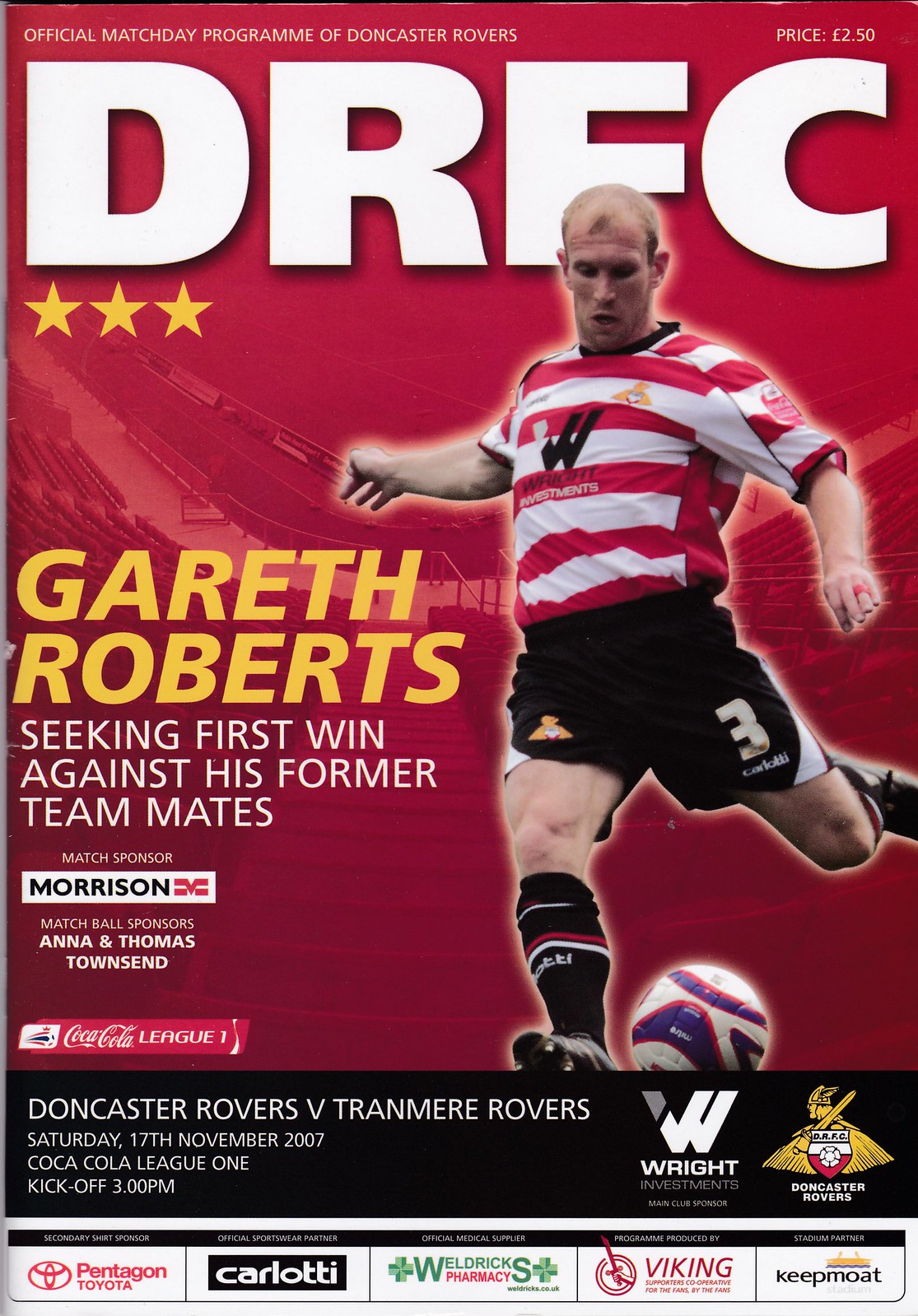The cover of the magazine or sports program features a dynamic scene with a red background dominating the top four-fifths of the page. An aerial view of a soccer stadium from the audience's perspective adds depth beneath the overlaying elements. Prominently positioned is a photograph of a muscular man with reddish-blonde hair, dressed in a short-sleeved red and white horizontally striped jersey, black shorts with a gold number three, and black socks adorned with red and white stripes. He is poised to kick a blue, white, and red soccer ball, his right leg swung back in preparation.

At the very top of the cover, white text reads, “Official Match Day Program of Doncaster Rovers, Price £2.50, DRFC.” The large acronym "DRFC" sits above the player’s head, with three yellow stars positioned below the letter 'D'. On the left, in capital yellow letters, the player's name "Gareth Roberts" is featured, followed by a white subtext stating, "Seeking first win against his former teammates, Match Sponsor Morrison, Match Ball Sponsors Anna and Thomas Townsend." Below the main photo, there is additional information: "Coca-cola League, Doncaster Rovers V Tranmere Rovers, Saturday 17th November 2007, Coca-cola League One, kickoff 3 p.m.” The comprehensive design encapsulates the excitement and anticipation of match day.